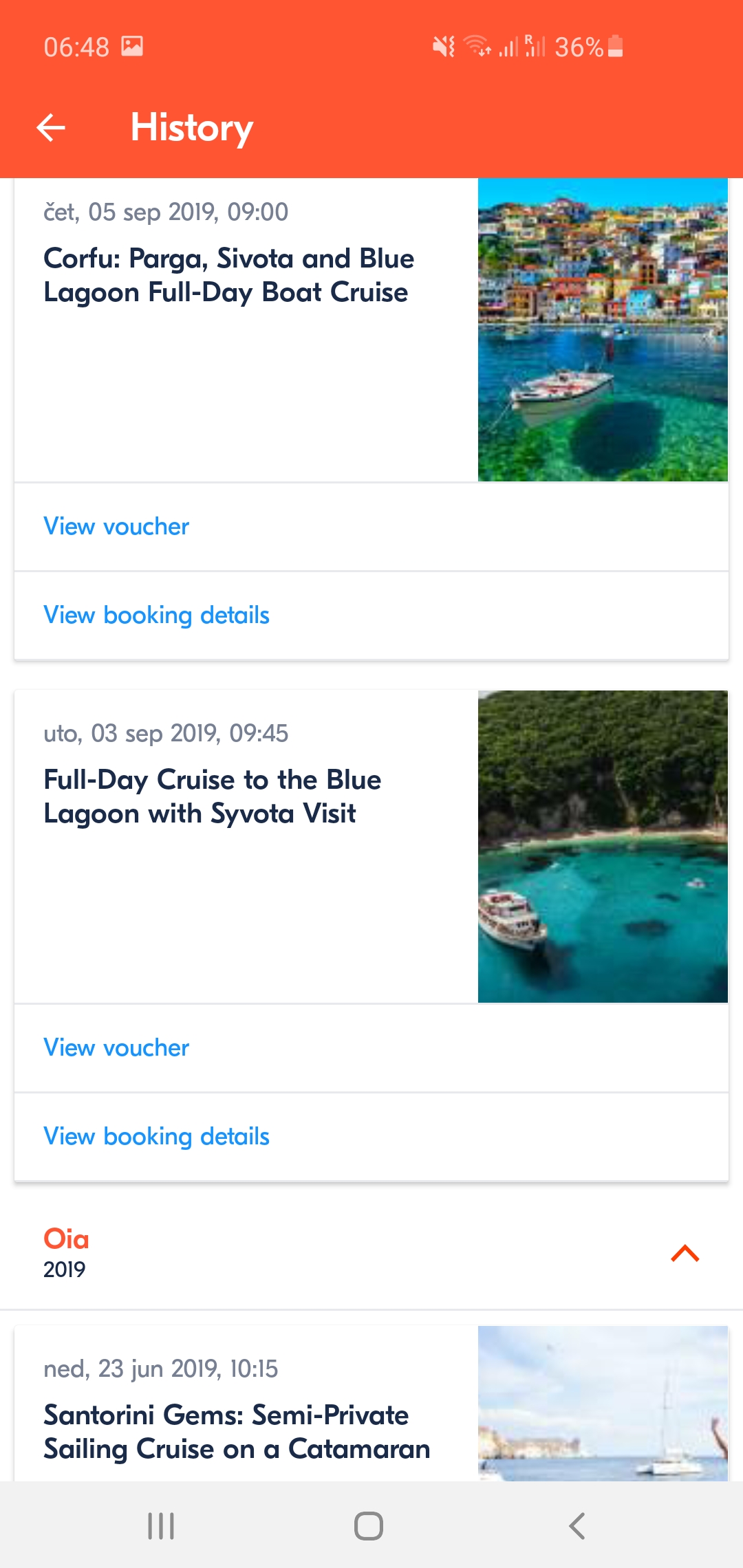Set against a clean white background, the image showcases a screenshot with a prominent red header at the top. In the upper left corner of the header, the time "6:48" is displayed in white text, while the bold white text "History" is centered below the header. The upper right corner of the header features icons for notifications, reception, and battery status, indicating that the battery is at 36%.

Beneath the red header, the screenshot displays an image of a picturesque city along a waterway, evoking a serene and captivating atmosphere. To the left of the image, the text reads "5th of September, 2019, 9 o'clock" in a legible font. Below this, in dark bold text, the details of a scenic adventure are highlighted: "Corfu, Parga, Sivota, and Blue Lagoon Full Day Boat Cruise." This is followed by the call-to-action phrases "View Voucher" in light blue text and "View Booking Details" beneath it.

The lower section of the screenshot contains a secondary image of boats on water and a beach, enhancing the allure of the travel experience. To the left of this second image, the text describes another engaging activity: "Full Day Cruise to the Blue Lagoon with Sivota Visit."